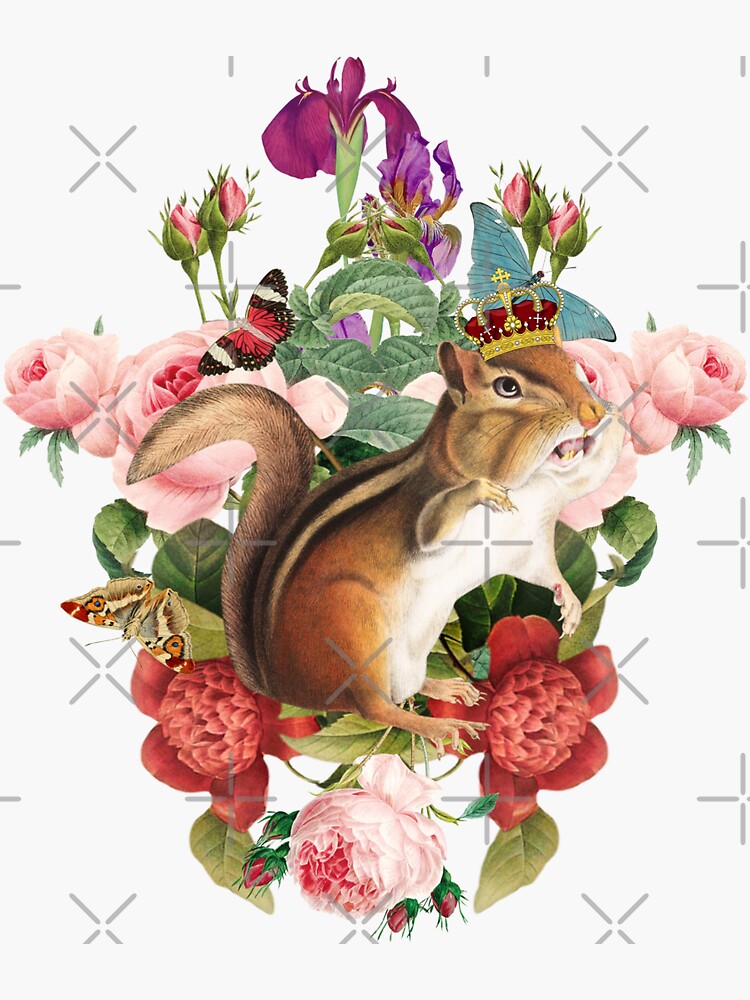The image is a rectangular, greeting card-style illustration with a light white background decorated with subtle gray X's and an intricate gold watermark. At the center of the image is a brown chipmunk with a white underbelly, wearing a regal gold and red crown adorned with a star on top. The chipmunk is positioned sideways, looking up to the top right with its mouth open, revealing its bottom teeth and its right eye visible. Surrounding the chipmunk is an elaborate bouquet featuring various flowers: pink carnations, red roses, budding red flowers, and greenery. There are also strawberries interspersed among the flowers and a butterfly situated on the left side, with an additional red butterfly at the top left. Towards the top of the image, there are delicate purple and dark purple floral designs, adding to the ornate, whimsical nature of the scene.